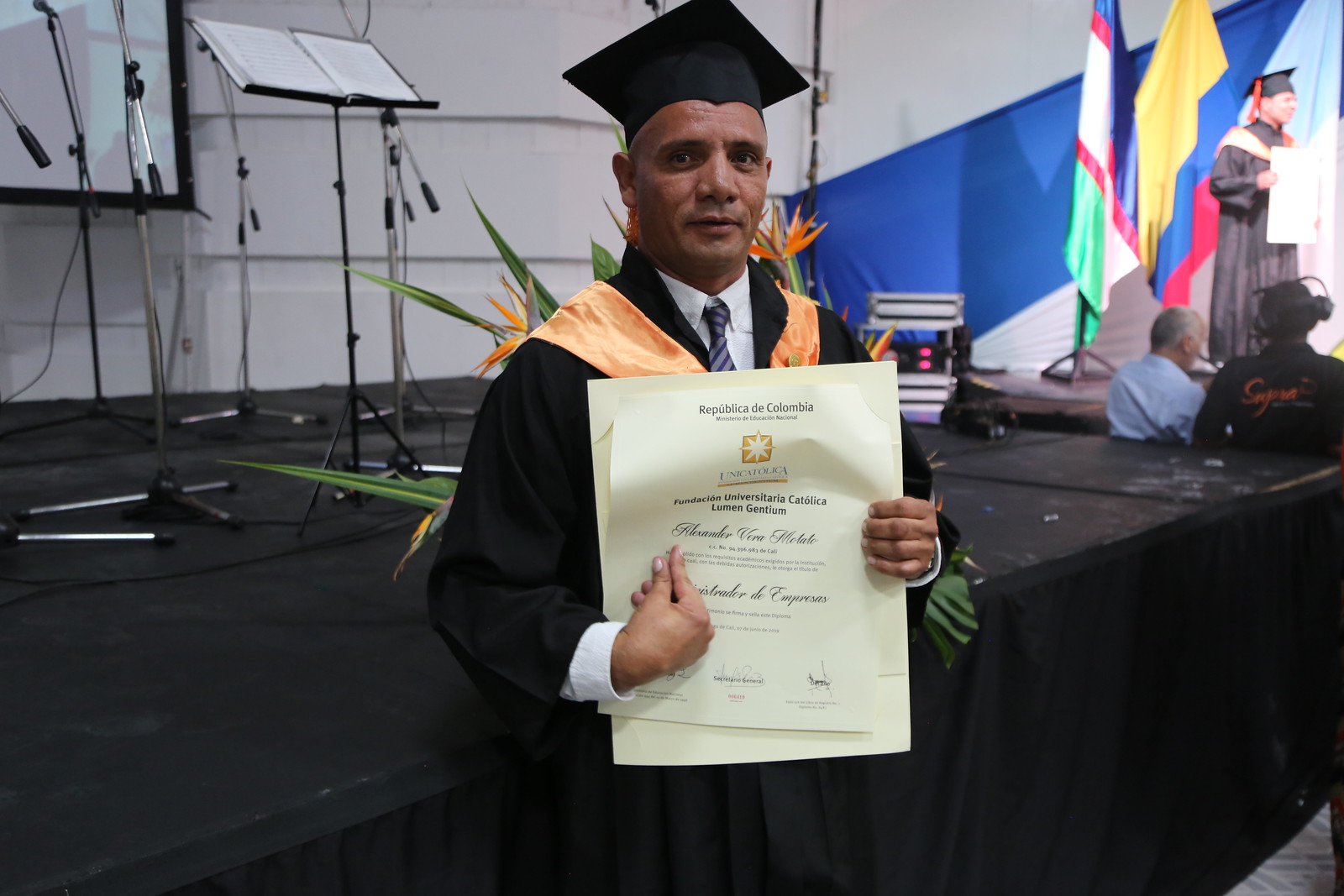A man, identified as Alex, stands at the center of the image, marking a moment of achievement at his graduation ceremony. He is clad in a black cap and gown, complemented by a white collared shirt and a blue tie underneath. Draped over his shoulders is a distinguishing yellow-orange sash. Alex is holding up a diploma with his left hand, showcasing the text "Republica de Colombia" prominently written on it. His right hand points toward what is likely his name on the diploma in a somewhat stiff manner.

Set against a black stage, the backdrop features several elements of a ceremonial scene: a music stand with papers, microphone stands, and equipment scattered throughout. Over Alex's right shoulder, you can discern heads and backs of other individuals, along with what seems to be another stage reflected in what appears to be a mirror in the upper right. On this secondary stage, another graduate is visible, similarly dressed in a cap and gown, but adorned with a red tassel and framed by colorful flags. Behind Alex, there is also a suggestion of floral arrangements like Birds of Paradise contributing to a festive atmosphere.